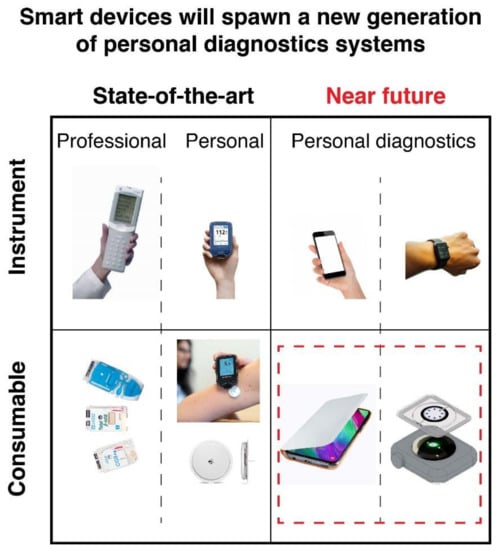The image is a detailed infographic on a white background outlining the evolution of smart devices in personal diagnostics. At the top, black text proclaims, "Smart devices will spawn a new generation of personal diagnostic systems." Beneath this heading, a large square is subdivided into four smaller squares, divided by a dotted line into two main columns: "State-of-the-art" in black and "Near Future" in red.

On the left side, the y-axis is labeled vertically with "Instrument" above and "Consumable" at the bottom. The "State-of-the-art" section is bifurcated into "Professional" and "Personal." The "Professional" box features an individual holding up a device that appears to be used in a clinical setting. Adjacent to it, under "Personal," a hand is shown holding a smaller gadget, suggesting current consumer-grade health tech.

The "Near Future" section anticipates advancements in personal diagnostics. One square displays a hand clutching a smartphone with a white screen, presumably for health-tracking apps, and another shows a wrist wearing a smartwatch. The bottom-right quadrant labeled "Consumable" includes various devices, such as a woman applying a device to her arm, likely for tracking metrics like glucose levels or blood pressure. Scattered within are blue-and-white gadgets, a small device with a white surface, and an iPad-like monitor displaying red and green indicators.

This infographic emphasizes the potential leap from current diagnostic tools to advanced smart devices aimed at enhancing personal health monitoring.